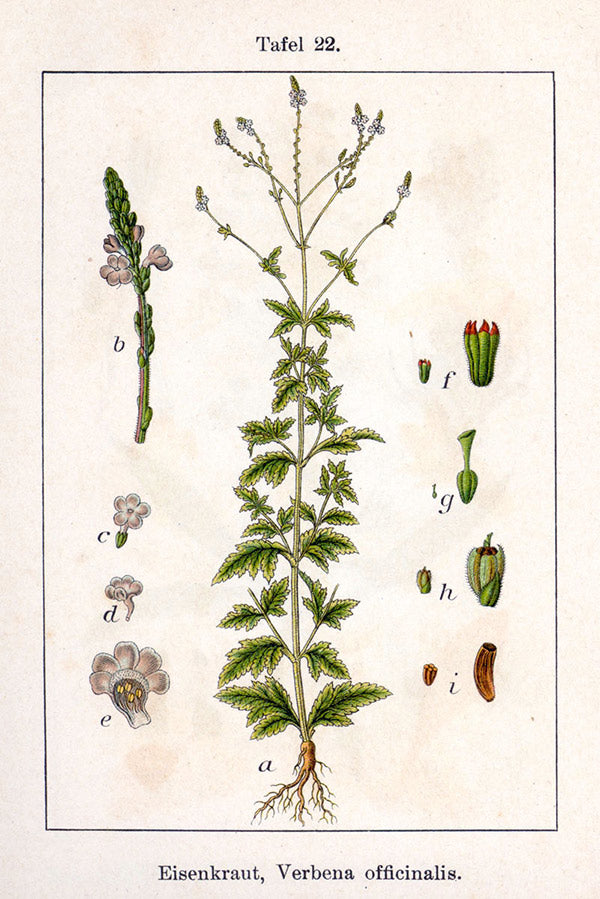This is an educational poster that provides an in-depth description of the plant Verbena officinalis, commonly known as Eisenkraut. The detailed botanical illustration, set against a white background, prominently features the complete structure of the plant labeled as 'A' in the center. This includes its long green stems, leaves, and a display of pink flowers positioned at the top. The labeled diagram extends from the root system at the bottom, growing tall to the bloom at the apex.

Surrounding the central illustration are additional graphical insets, each labeled from B to I, depicting various parts of the plant in greater detail. This allows viewers to examine parts that might not be clearly visible in the main structure, including leaves, stems, roots, and flowers. The overall design emphasizes scientific accuracy and educational value, with the main title "Toffle 22" positioned at the top, along with the plant’s Latin name and common name, enhancing the informative nature of the poster. The use of green and red hues in the illustrations adds to the visual clarity and appeal.